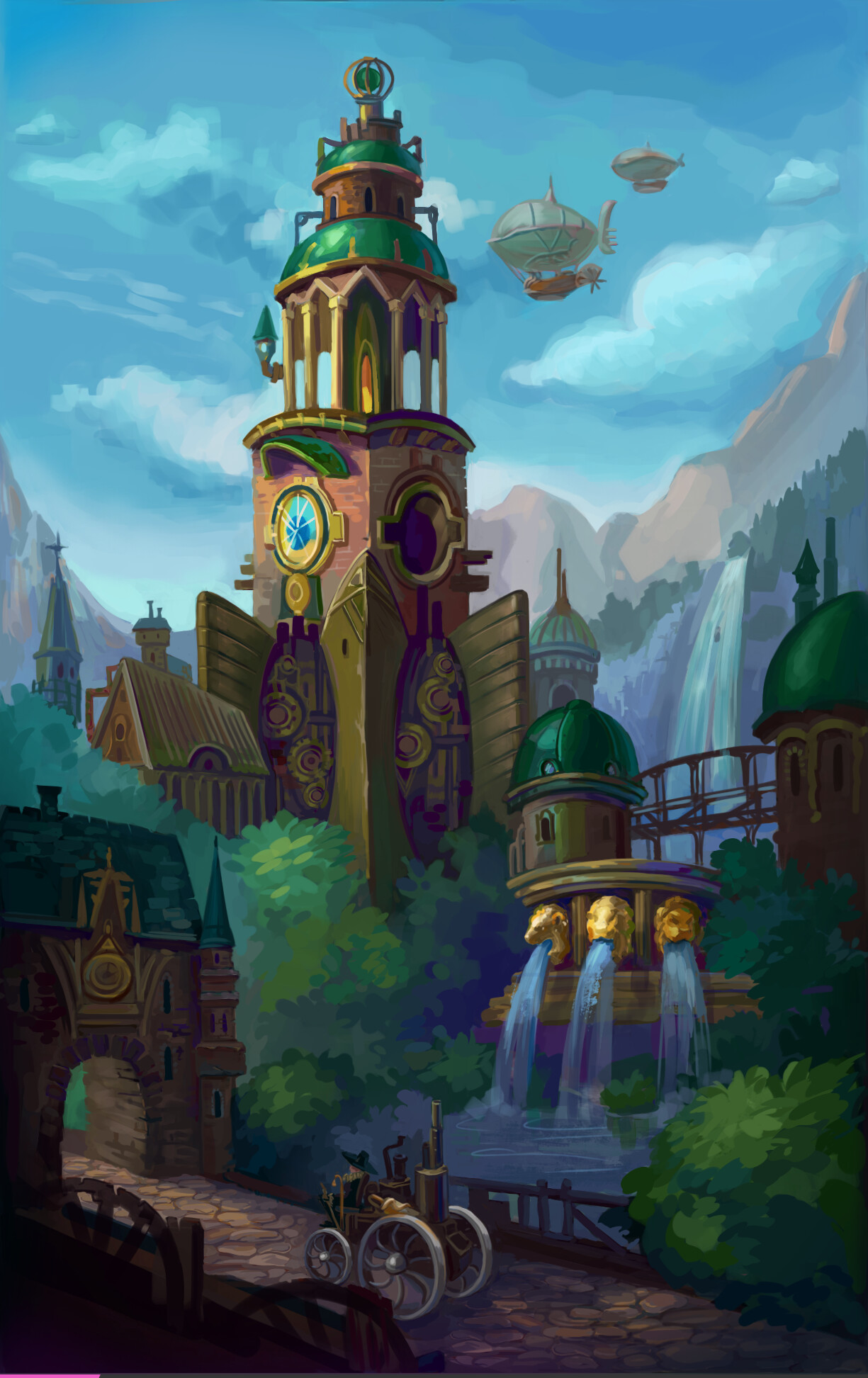This detailed painting, possibly a computer-generated artwork, depicts a vibrant steampunk world, set amidst an outdoor, mountainous region. Central to the image is a towering, steeple-like castle, doubling as a clock tower with vivid clock faces on each side and adorned in brass accents. The roofs, painted in a patina copper green, contrast against the dominant purples throughout the scene. A long flame seems to emanate from the top of the tower, which is designed like a gazebo or balcony.

Below the tower is a section resembling a church, embellished with intricate gears. Situated in the foreground are two bridges, one directly ahead and the other slightly behind, each flanked by lion-headed fountains that spill water into a serene lake. Crossing one bridge is a steam-powered buggy, adding to the steampunk aesthetic.

The sky is a mix of blue and cloudy hues, populated by fantastical airships akin to hot air balloons. The entire scene is nestled within a natural backdrop of dark green forests and brown mountains, with a waterfall cascading down the right side, adding an enchanting feel to the overall depiction.